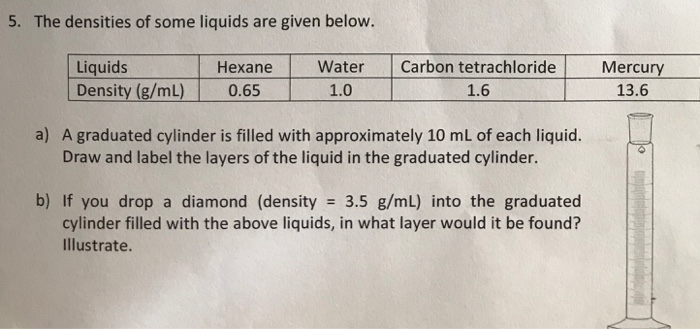Caption: 

An image showing Question 5 from a chemistry test printed on slightly grayed paper. The question provides the densities of various liquids: hexane, water, carbon tetrachloride, and mercury. Part A of the question asks students to fill a graduated cylinder with approximately 10 milliliters of each liquid and then draw and label the layers based on their densities. Part B of the question poses a challenge: determining which layer a diamond—having a density of 3.5 grams per milliliter—would settle into when dropped into the graduated cylinder filled with these liquids.